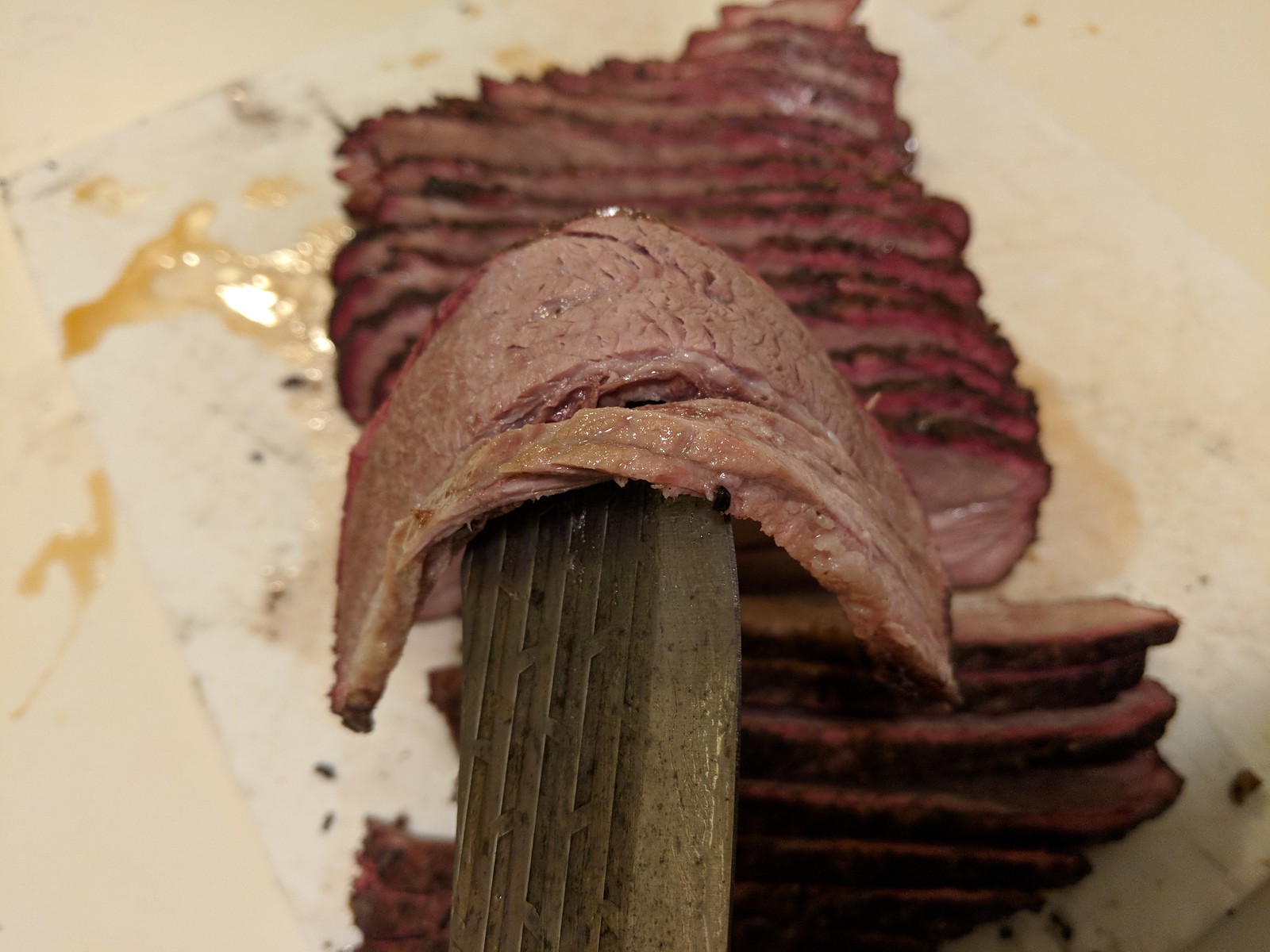This photograph showcases a large, pewter-colored butcher knife holding a juicy slice of smoked beef brisket in the foreground. The slice of brisket, featuring an appetizing pink smoke ring indicating perfect smoking, is draped over the knife, emphasizing its tenderness. Behind this, on a white cutting board, lies a tantalizing spread of thinly sliced brisket, likely about two dozen pieces. The brisket appears exceedingly juicy, with visible fat and meat juices pooling around the slices, enhancing their mouth-watering appearance. The setting evokes a restaurant or buffet atmosphere, where the brisket has been meticulously prepared and served.